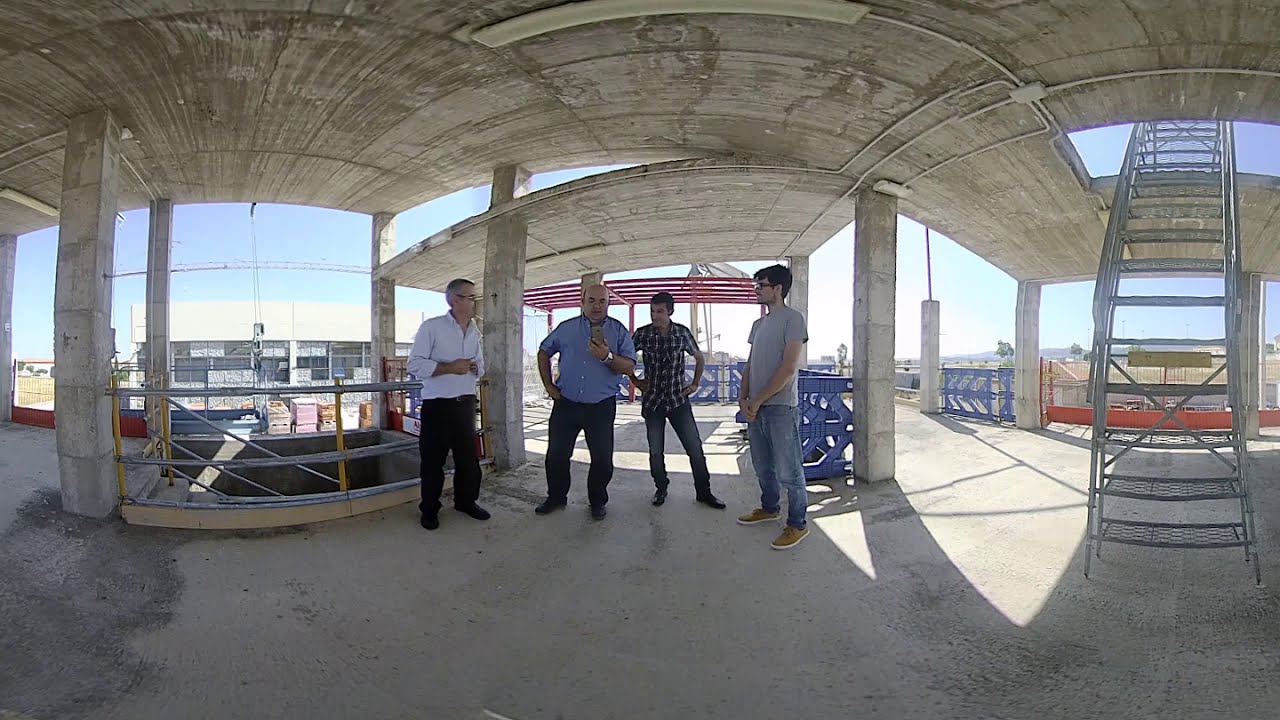In this fisheye photograph taken from inside an under-construction building, four men are standing closely together on a freshly poured light gray cement floor. Casting shadows as they stand under an overhead arched ceiling, they are positioned centrally in the image, flanked by the open walls through which the bright blue sky and surrounding skyline are visible. 

To the left of the image stands an older man, possibly in his 50s, wearing a white open-collared shirt and black trousers. He has gray hair, wears glasses, and stands near a stairwell going downward, potentially to stadium seating. Next to him, looking at his phone, is a middle-aged man in his 40s, wearing a short-sleeved blue shirt tucked into black pants. He is somewhat balding and stands facing forward.

Next to the man with the phone is a younger individual in his late teens or early 20s. This young man, with dark hair and wearing a plaid short-sleeve shirt with blue jeans, stands with his arms akimbo, hands on his hips. Finally, on the rightmost side of the group is another young man, also in his late teens or early 20s. He is wearing a light gray t-shirt, stonewashed jeans, and tan sneakers, standing relaxed with his arms loosely at his sides, slightly in front of him.

In the background, bright sunlight streams through the structure, illuminating the surroundings while the men remain in shadow. To the right of the image, a metal staircase ascends to the second level, where thin, freshly poured cement forms the flooring, supported by rectangular columns of the same material.